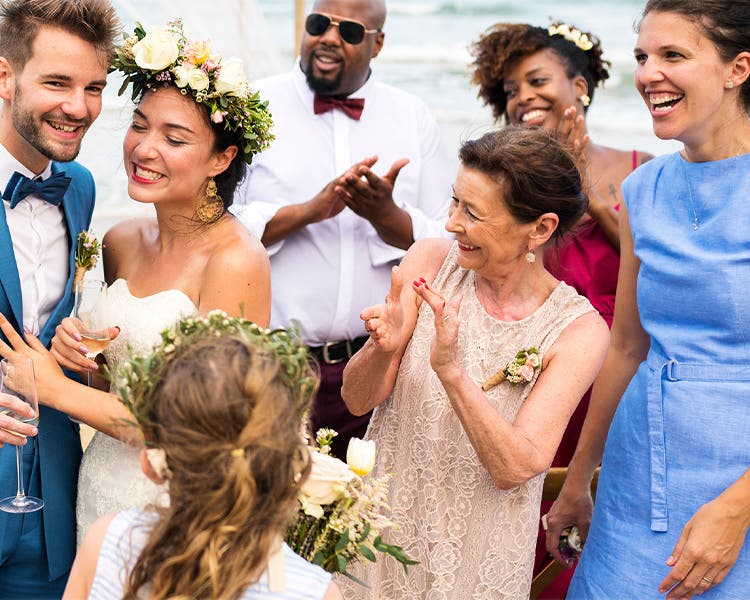This candid wedding celebration photograph showcases a joyous moment with the bride and groom surrounded by their loved ones. The groom, dressed in a cyan blue suit with a white shirt and dark blue bow tie accented with cyan, holds a champagne glass, his light, spiky brown hair, beard, and mustache adding to his debonair look. The bride, close beside him with one hand on his chest and the other holding a champagne glass with a slight orange tint, radiates happiness. She is adorned in a white, shoulderless, strapless dress and a floral crown woven with white, orange, and pink flowers, with delicate green leaves peeking through.

Behind and around them, the guests are immersed in the celebration. The immediate foreground captures the back of a probable bridesmaid's head, her dirty blonde hair cascading down, adorned with a floral crown matching the bride's, hinting at her role in the ceremony. A bouquet of white flowers with orange and yellow accents is clasped in her hands.

To the right of the bride stands an elderly woman, likely the bride’s mother, in a tan shift dress with her hair elegantly pinned up and a corsage of pink flowers fastened with brown twine on her wrist, poised to clap with her hands together, her nails painted in shades of red and pink. Next to her, a woman in a light blue shift dress beams warmly, displaying a full smile.

In the background, an African-American couple adds to the scene’s vibrancy. The man sports a white shirt paired with a red bow tie, golden-rimmed sunglasses, and a distinguished bald head with a goatee. The woman, donning a red sundress adorned with golden earrings and a small hair clip, smiles broadly. The sunny outdoor setting bathes everyone in a warm glow, encapsulating the love and joy of this special occasion.